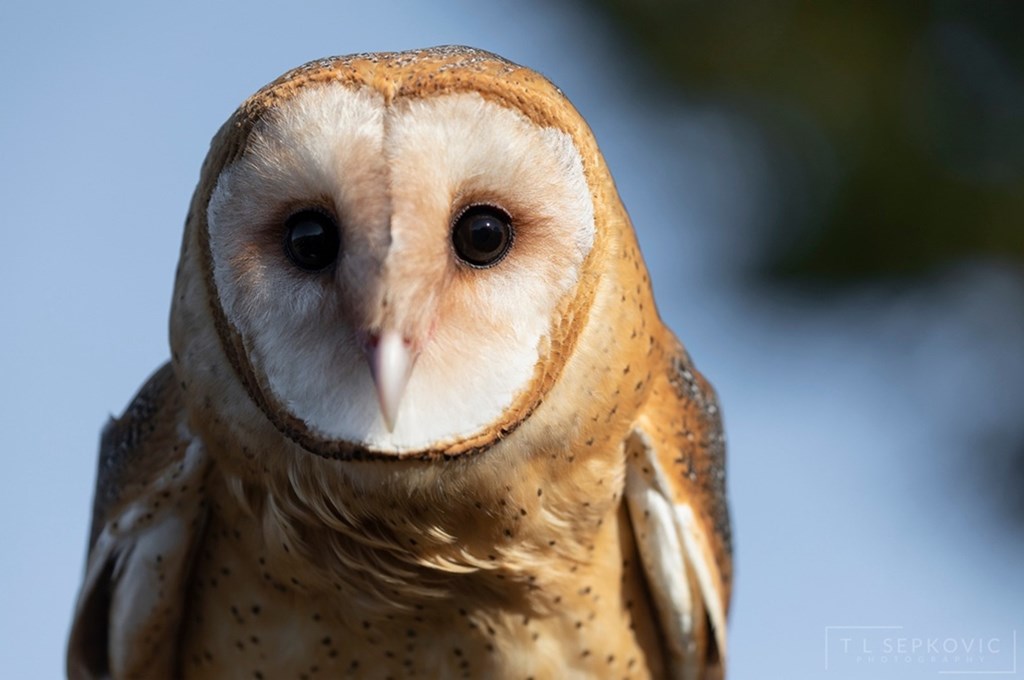This photograph captures a close-up of a young owl with a heart-shaped, white face and dark, black eyes, staring directly at the camera with an intense, curious gaze. The owl's head and upper body dominate the image, with feathers around its eyes and head displaying a blend of yellowish-orange and brown hues. Its sharp beak points straight ahead, enhancing the penetrating look. The owl’s breast features light yellow feathers speckled with numerous black dots. The top of its wings show darker brown feathers, almost black, while the underside is whitish. The focus on the owl creates a beautifully blurred background of blue sky, which shifts to a greenish hue in the upper right corner, suggestive of blurred foliage. The photograph appears to be set against this soft backdrop, and although the owl is perched and still, its depiction brims with life. In the bottom right corner of the image, a watermark reading “T.L. Sepkovic” is visible.